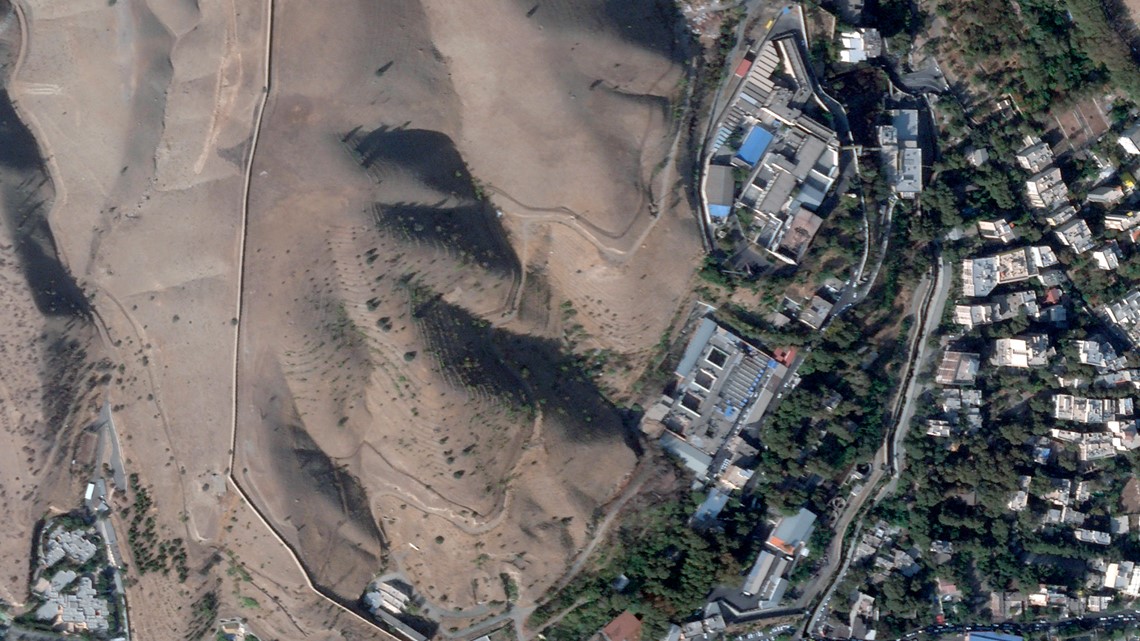The image is a contemporary satellite or aerial photograph resembling a topographical or Google Earth map. The left two-thirds of the image are dominated by a sandy, light beige terrain, interspersed with hints of green, likely indicating sparse vegetation or clumps of trees. This area features undulating sandy hills and a prominent road that runs roughly from the upper middle section diagonally downward to the right. The right third of the image transitions into a more developed landscape, depicting a community. Here, the tops of numerous houses are visible, set against a backdrop of more densely clustered trees, suggesting a relatively new or up-and-coming area rather than a fully developed city. The roofs of the houses form a pattern, and the community is crisscrossed with roads, though specific details of the houses are indiscernible. This bird's-eye view captures the stark contrast between expansive desert terrain and a burgeoning residential area.